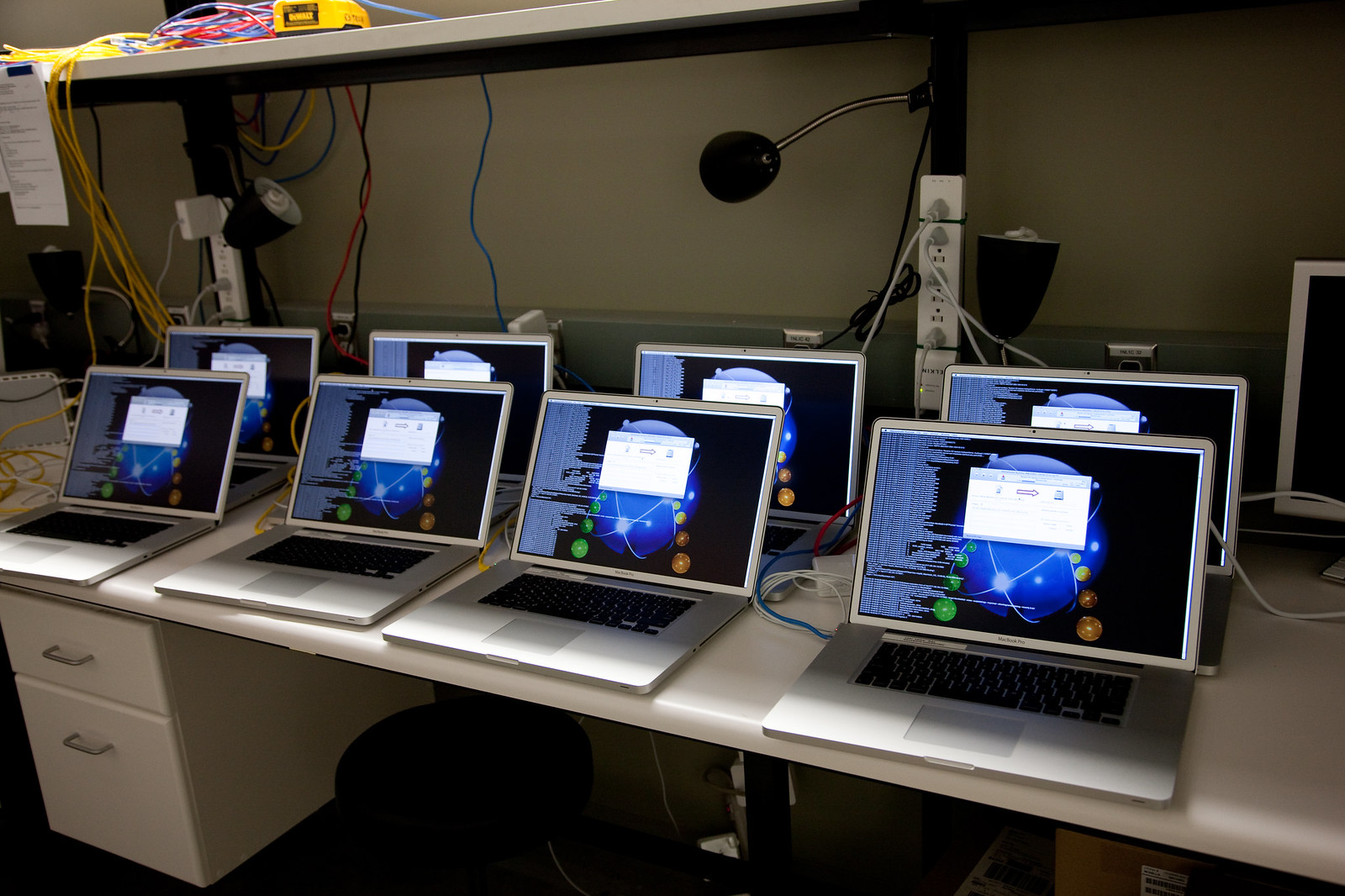This photograph captures a bustling laptop service area set within a cubicle-like office space. Positioned on a long, white workbench, there are eight silver laptops arranged in two neat rows of four, all displaying a diagnostic screen with a blue globe, green and orange circles, and a white text box overlaying the globe. The keyboard area of each laptop is black, while the touchpad area is silver. 

The workbench is flanked by two white filing cabinets on the left and some boxes on the right, all beneath a secondary white shelf. A black stool is tucked under the bench near the filing cabinets. The rear shelf, mounted above the work surface, supports numerous yellow, red, and blue cables swooping down towards the laptops, along with black zip-tied power strips populated with various power cords.

Additionally, two adjustable gooseneck lamps are secured to black vertical bars running down from the shelf, providing flexible lighting over the work area. The scene also features the bottom part of a yellow drill and scattered white papers hanging off the shelf. This setup indicates a highly organized and active environment, likely engaged in preparing or repairing these laptops for distribution or further use.